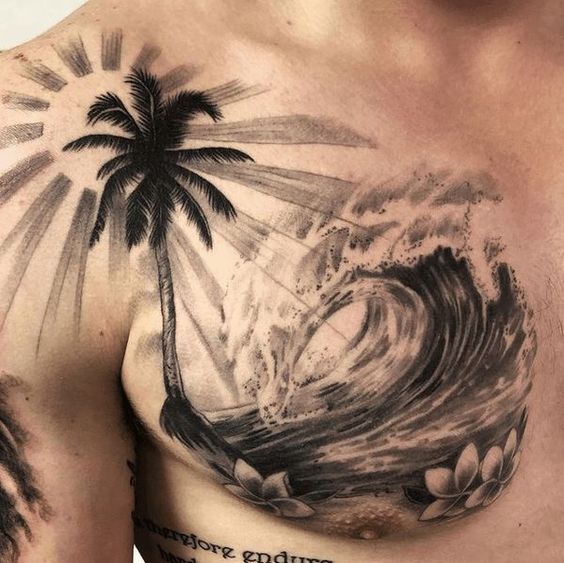The image depicts a detailed black and white tattoo covering the right shoulder, pectoral, and upper arm of a muscular man. Centered prominently on the right shoulder is an open sun with radiating rays, partially obscured by a tall, thin-trunked palm tree. The palm tree extends from his shoulder down to his chest, where its roots blend seamlessly into a dynamic wave, curling back toward the palm tree with distinct white caps. Interwoven with the waves are several plumeria flowers, with one situated on the left and two on the right. Near the bottom of the design, close to the man's ribcage, is some partially visible black lettering, adding an additional layer of mystery to the intricate tattoo. The entire composition is well-balanced, perfectly following the contour of his developed pectoral muscles and shoulder.